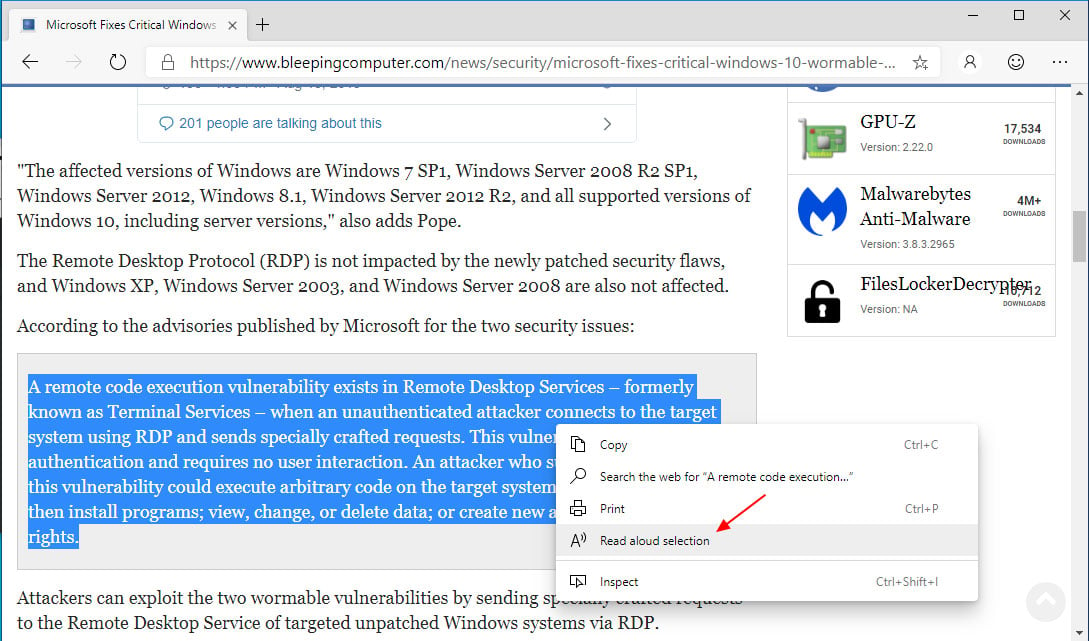In this image, we see a web page from bleepingcomputer.com. The browser tab at the top reads, "Microsoft Fixes Critical Windows Issue," indicating the topic of the page. Below the web address bar, a paragraph outlines the details of the article. It mentions that the affected Windows versions include Windows 7 SP1, Windows Server 2008 R2 SP1, Windows Server 2012, Windows 8.1, Windows Server 2012, and all supported versions of Windows 10, including their server versions. It also specifies that the Remote Desktop Protocol (RDP) is not impacted by the newly patched security flaws and that earlier versions like Windows XP, Windows Server 2003, and Windows Server 2008 are also unaffected, according to advisories published by Microsoft regarding two security issues.

Further down, another paragraph begins but is partially obscured by a pop-up box. This paragraph describes a remote code execution vulnerability in Remote Desktop Services, formerly known as Terminal Services, where an unauthenticated attacker could connect to the target system using a specially crafted RDP request. The pop-up box contains an arrow pointing to a "read aloud" section, further obstructing the text.